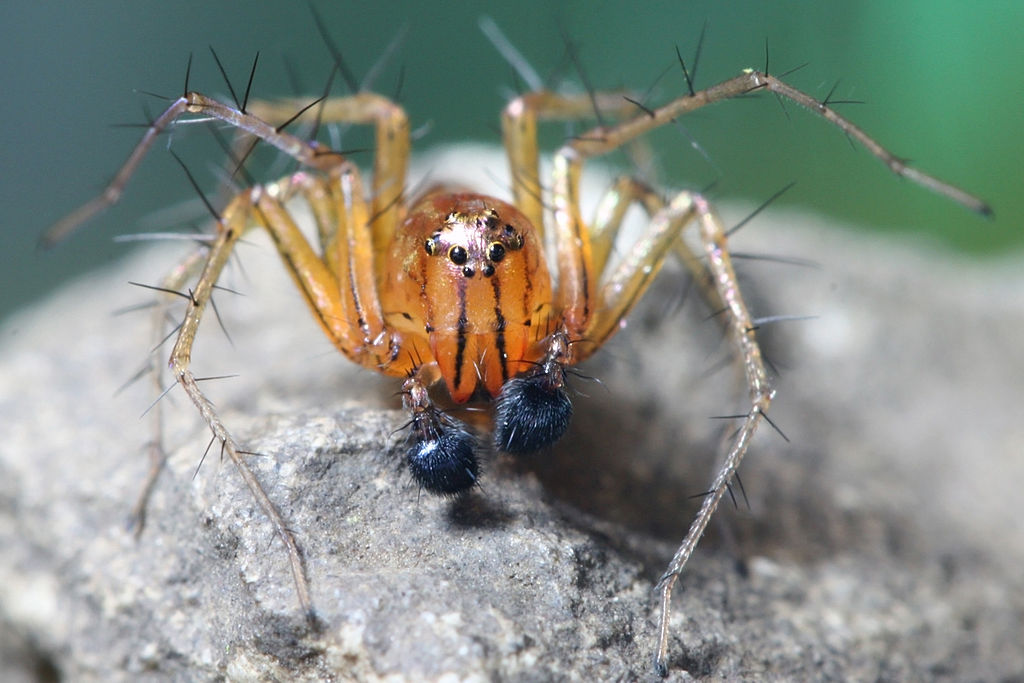This highly detailed, color photograph features an extreme close-up of a golden-orange spider perched on a granite-colored rock. The image is in landscape orientation, allowing the spider to fill most of the frame. The background is blurred with hints of green, keeping the focus squarely on the spider. The spider’s eight legs start as translucent amber near the body, fading to almost clear white at the tips. Each leg is adorned with long black bristles, clustered at the joints. The spider's body showcases intricate black markings, particularly down its front and along the sides of its legs. Its face, the sharpest area of the image, reveals approximately eight black, bead-like eyes staring directly at the camera, giving the spider a somewhat eerie appearance. Prominently visible are two fuzzy, black, boxing-glove-like appendages near its mouth, adding to its distinctive visage. The photograph's high resolution and sharp detail, especially of the spider's face, evoke a quality akin to that of professional nature photography, reminiscent of an image one might find in an insect or National Geographic publication.